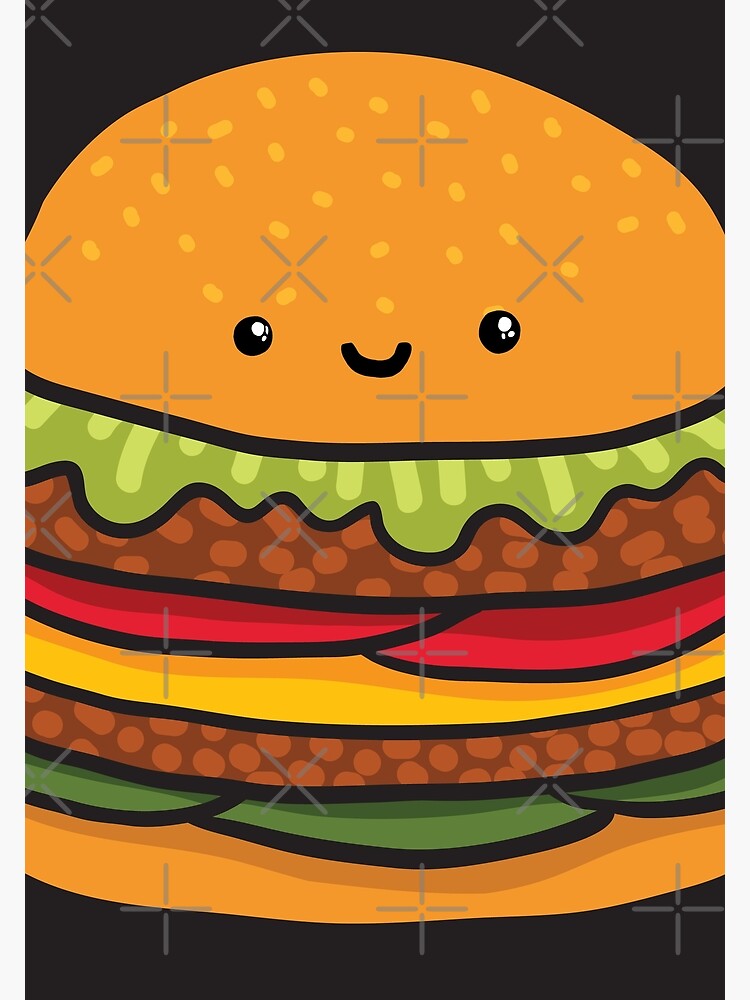This playful, cartoon-style drawing depicts a hamburger set against a black background. The sesame seed top bun is dome-shaped, orange in color with yellow seeds, and features two black eyes adorned with white reflections, as well as a small, curved mouth, giving it a cute, smiling face. Below the cheerful bun, there's a layer of fresh green lettuce. Following it is a juicy brown beef patty dotted with light brown specs. Next comes a pair of red tomato slices, a layer of yellow cheese, and another brown beef patty speckled with brown dots. Just beneath this patty lies a trio of green pickles. Finally, the ensemble sits atop the bottom bun, completing the whimsical and appetizing image reminiscent of a Big Mac.